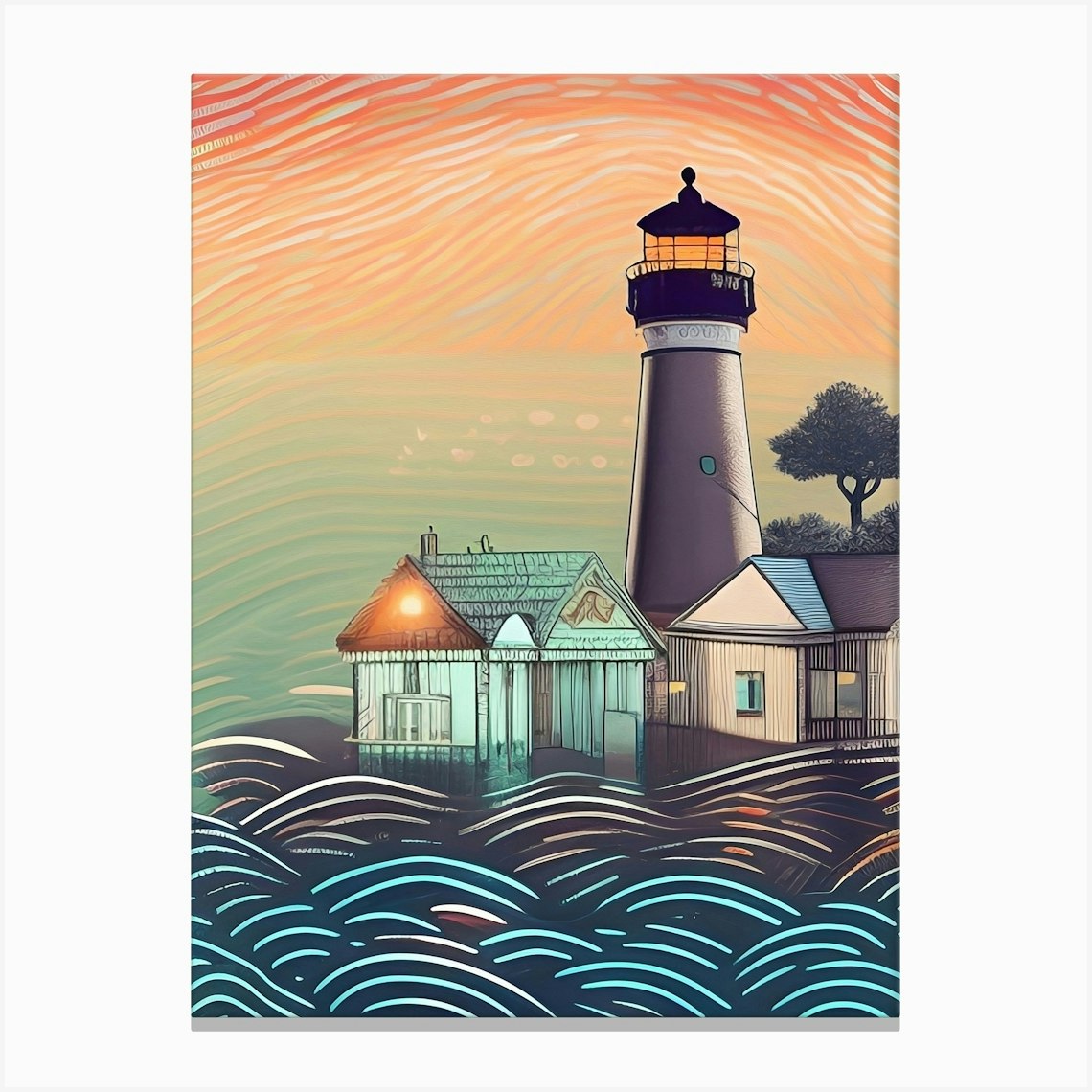This artist's painting portrays a vibrant outdoor lighthouse scene amidst nature. The foreground is characterized by dynamic, arching waves, almost resembling a plowed field. The composition features a prominent red lighthouse with an illuminated black turret casting an amber glow. Flanking this lighthouse are buildings: one with a red awning and white shingles, another painted pink, and a third one in light teal. The scene is enriched by a backdrop of lush forest and a singular silhouetted tree. The sky is depicted with a striking, almost turbulent blend of orange, yellow, and light blue ripples, adding a dramatic intensity to the overall mood. The artist’s use of color and abstract forms makes the scenery feel both surreal and compellingly alive.